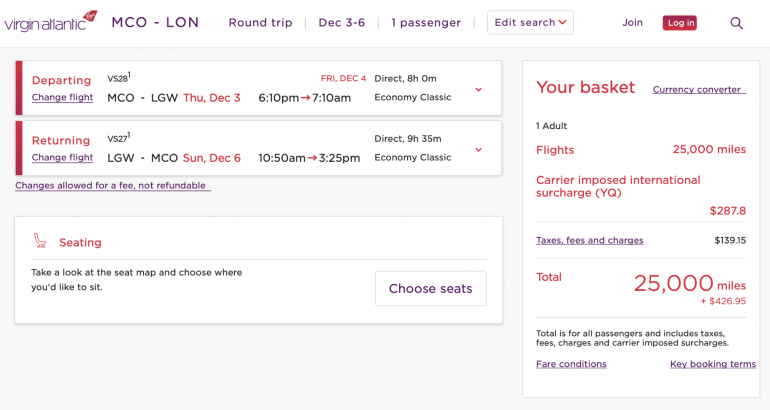**Virgin Atlantic Round Trip Itinerary: MCO to LGW**

This image showcases a detailed Virgin Atlantic itinerary for a round trip from Orlando International Airport (MCO) to London Gatwick Airport (LGW). The travel dates are from Thursday, December 3rd, to Sunday, December 6th. 

### Flight Details:
- **Outbound Flight:** 
  - MCO to LGW
  - Thursday, December 3rd
  - Time: Displayed
  - Class: Economy
  
- **Return Flight:** 
  - LGW to MCO
  - Sunday, December 6th
  - Time: Displayed
  - Class: Economy

### Booking Information:
- **Passenger Details:** 
  - One Adult
  - Editable Search Box with Red Checkmark
  - Option to Join or Login
  
- **Flight Options:**
  - Departing and Returning flight details are highlighted in red
  - Option to Change Flight is highlighted in purple

### Seat Selection:
- **Seating:**
  - Option to View and Choose Seats from a Seat Map
  - Seating information in red
  - Choose Seats button displayed in purple
  
### Fare and Charges:
- **Cost Breakdown:**
  - 25,000 Miles for Flights
  - Carrier-imposed International Surcharge in red
  - Taxes, Fees, and Total Amount in dollars
  - Total Miles and Total Payable Amount
  
- **Additional Information:**
  - Fare conditions and key booking items
  - Change allowed for a fee, non-refundable (highlighted in purple and underlined)

### Auxiliary Options:
- **Currency Converter:** Available in purple
- **Your Basket:** Displayed on a right-hand vertical box in green

The image presents essential details for managing the flight reservation, including options for changing flights, seat selection, and viewing fare conditions.